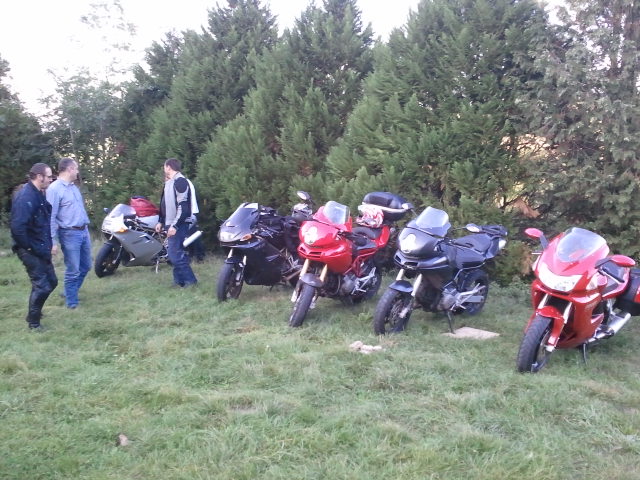This hazy daylight outdoor photograph captures a detailed scene of five modern motorcycles parked in a row on a green lawn, viewed from a three-quarter angle. The lineup consists of a red motorcycle on the far right, followed by a black one, another red one at the center, another black one next to it, and a gray motorcycle in the furthest background. Three white men are positioned on the left side of the image, with two walking into the frame. One of these men is dressed in blue overalls, while the other sports denim jeans and a blue shirt. A third man stands about four feet in front of them, wearing a motorcycle jacket and pants, with his head turned toward the gray motorcycle. The background features a line of evergreen trees under an overcast sky, and the foreground consists of cut grass. The photograph is slightly out of focus, adding to its non-professional feel. The motorcycles resemble sport scooters, with their lights possibly illuminated, creating an engaging, dynamic scene.